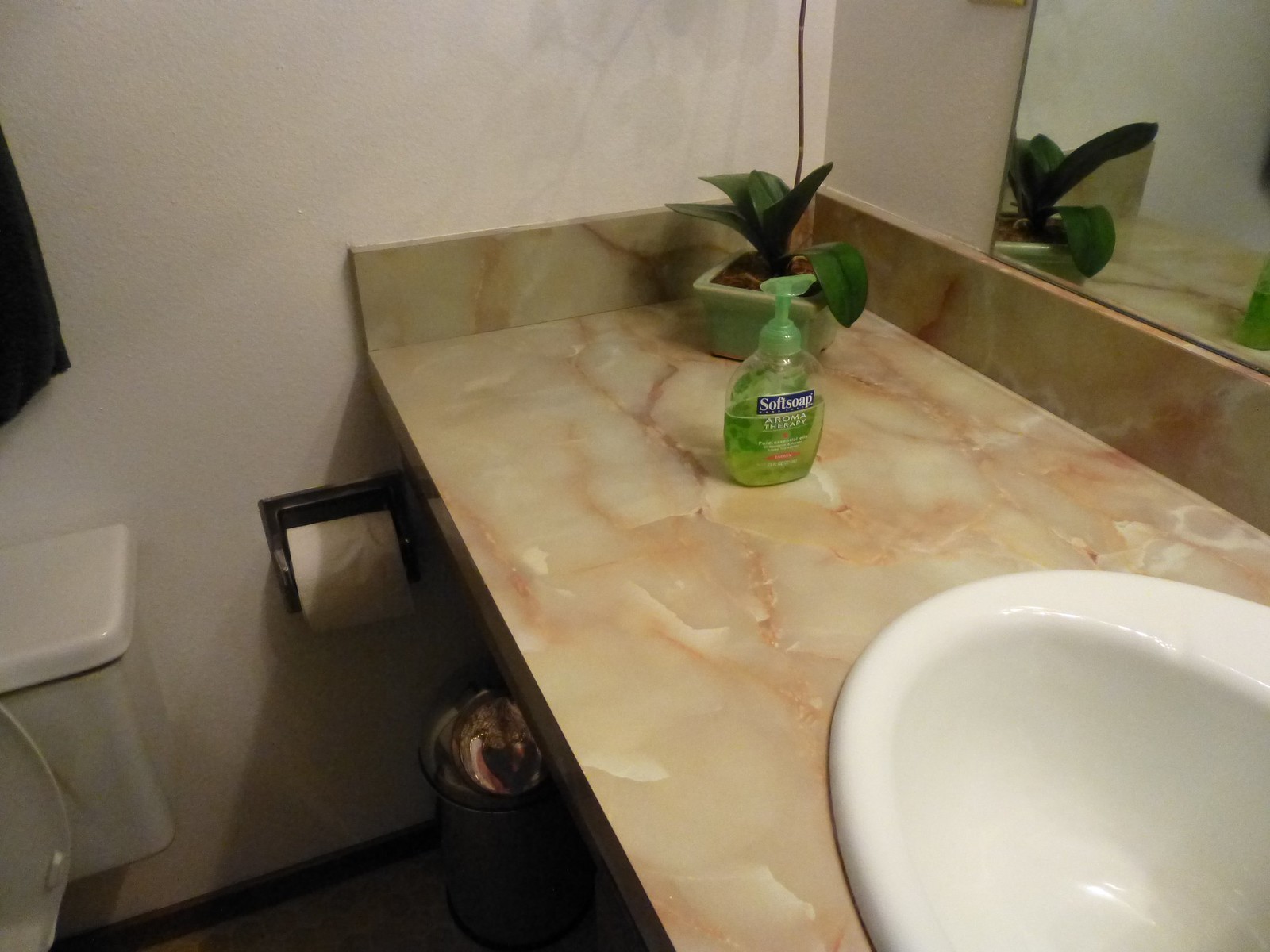A pristine white porcelain toilet with the seat up is the focal point of the bathroom. The back wall is painted a clean white, accentuated by a mirror in the top right corner, which reflects the interior of the bathroom. To the right of the toilet, a black metal fixture with silver arms secures a roll of white toilet paper. The wall also features a speckled pattern in light brown, white, gray, and other subtle hues.

A large green vase filled with soil sits prominently, housing several lush green leaves; one leaf bends over the edge, while three others stand upright. Next to the vase, a blue rectangular bottle labeled "Softsoap Aromatherapy" contains green liquid soap and has a pump at the top. This bottle is positioned on a countertop, which also appears to hold a trash bin underneath, partially visible.

The entire scene is illuminated, casting a shadow of the vase's leaves onto the far wall. A cable snakes down from the top of the image to the vase, adding a slight utilitarian touch to the overall aesthetic. Additional text on the Softsoap bottle is partially visible but unreadable from this vantage point, with some in white and a portion in red.